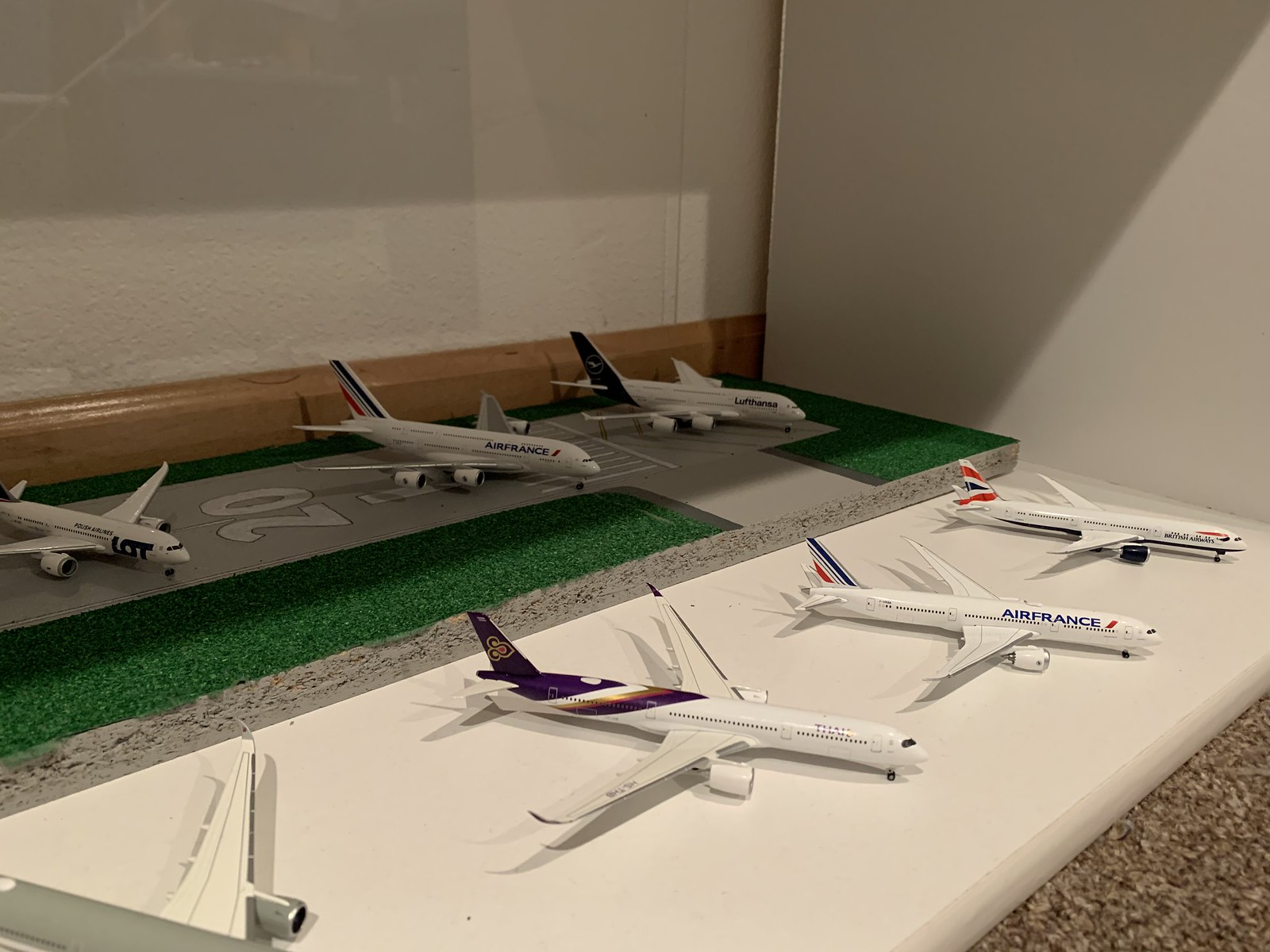The photograph showcases a detailed display of seven small model airplanes arranged in two rows, facing to the right. The scene is set against a white background with walls visible on the left and top right corners. The lower right corner shows a brown and tan table, and some light brown carpet is faintly visible. The back row consists of three model planes mounted on an elevated board designed to resemble a runway painted with green and gray colors, complete with white runway markings and numbers. Among these planes are models from various European carriers, including Air France, Lufthansa, and perhaps Turkish Airways, with Air France notably featuring white and blue colors. The front row, positioned on a lower shelf, includes four additional planes with diverse liveries such as a white and purple/gold design, another white Air France model, and white planes with red and blue stripes. The meticulous layout suggests a display that might be found at an airport or an aviation museum, capturing a miniature yet comprehensive essence of European air travel.